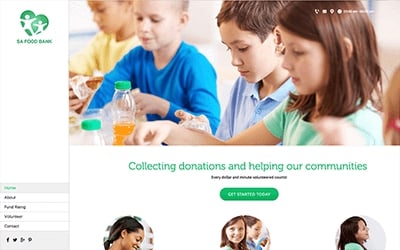This image showcases a website dedicated to a food bank. Located on the left side is a green heart-shaped logo. The main section features animated depictions of children, all seated at a table and engaged in eating and drinking. The group consists of four children: three boys sitting closely together and a girl positioned at the end of the table. Among them, one child is drinking from a juice bottle while another enjoys a sandwich. Beneath this scene, there's a prominent message stating, "Collecting Donations and Helping Our Communities," accompanied by a green "Get Started Today" button. Additional imagery includes a smiling African-American woman, who appears to be about 33 years old. There is also an image of a boy and girl seated beside each other. To the right, another woman with dark hair, estimated to be 35 years old, is pictured.